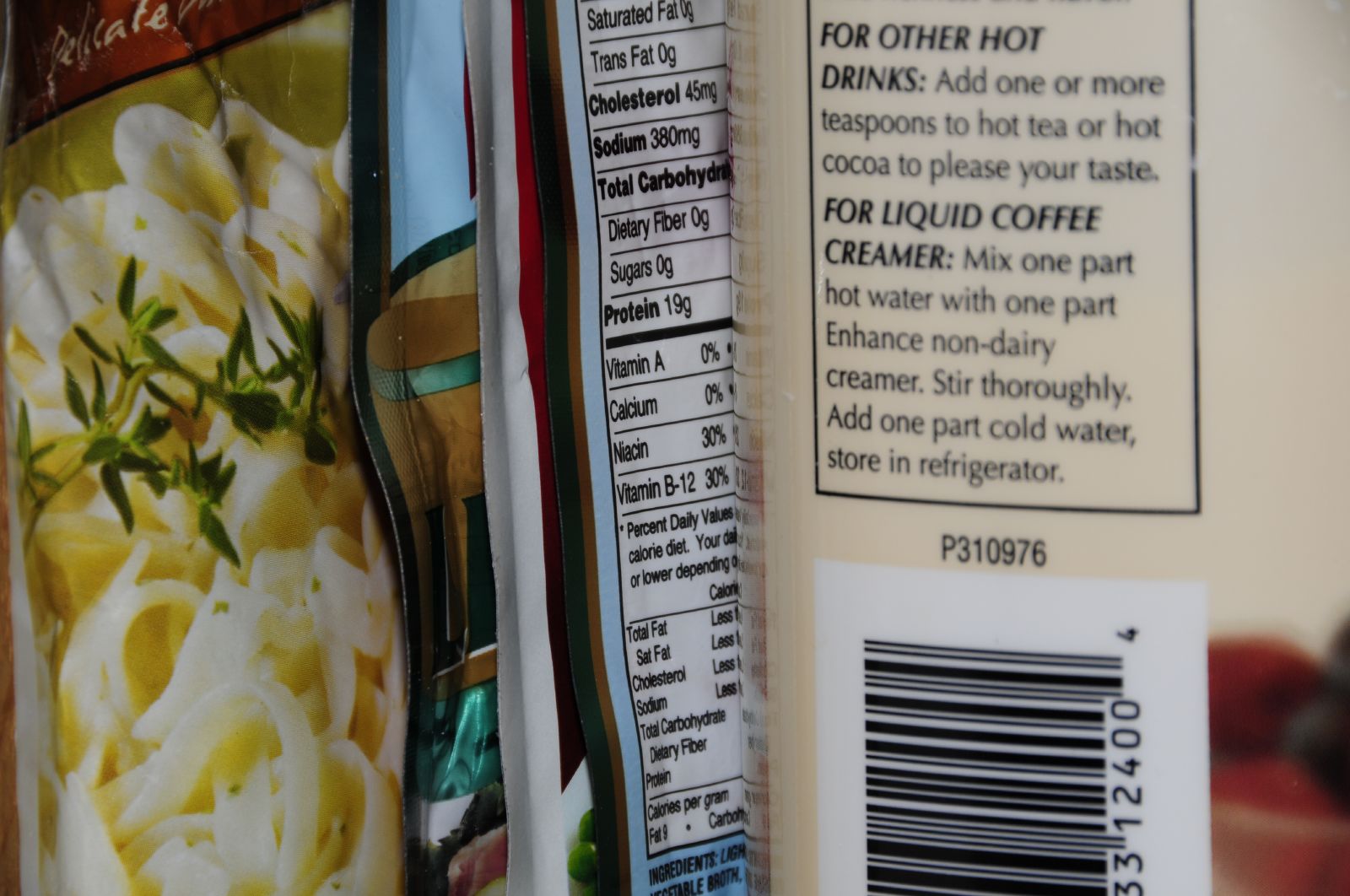The image showcases an assortment of food product packages arranged in a row. On the far right, there is a yellowish container featuring a UPC barcode at the bottom. The label on this container provides instructions for use, stating: "For other hot drinks, add one or more teaspoons to hot tea or hot cocoa to suit your taste. For liquid coffee creamer, mix one part hot water with one part enhanced non-dairy creamer, stir thoroughly, add one part cold water, store in refrigerator."

Moving towards the left, there are several bags of food items. Immediately to the left of the yellowish container, there is a bag labeled with nutritional information. Next to it, a blue and yellow bag is visible. On the far left, there is a bag with a red top that features an image of pasta, adorned with a hint of greenery.